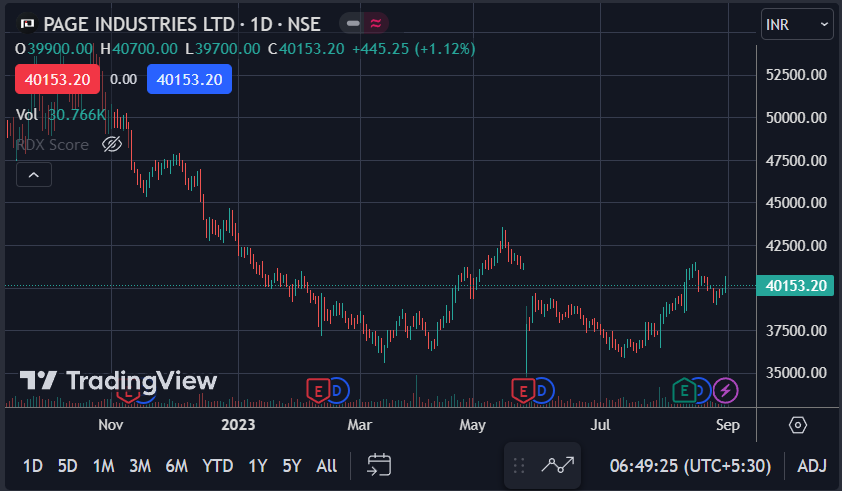Here is a cleaned-up and detailed caption for the image:

---

This is a screenshot of a graph depicting investment statistics for Page Industries LTD. The graph is presented on a Trading View platform, identifiable by its logo in the lower corner. The title of the graph is prominently displayed as "Page Industries LTD."

In the upper corner of the screenshot, there are two buttons: one red and one blue. The red button displays the figure "4153.20," and adjacent to it, there is a blank space showing "0.00." The blue button next to the blank space also shows the figure "4153.20."

The trading volume is marked at "30.766,000." The time frame of the graph spans from before November 2023 and progresses through March, May, July, and September. The trend line of the graph initially shows a decline, reaching its lowest point in March. Following this, there is a gradual upward movement until between May and June, where the trend begins to descend once more.

The graph itself is set against a dark blue background, with a vertical and horizontal grid providing a clear framework for visualizing the data. The platform allows for various options to customize the displayed information, enhancing the analytical experience for users.